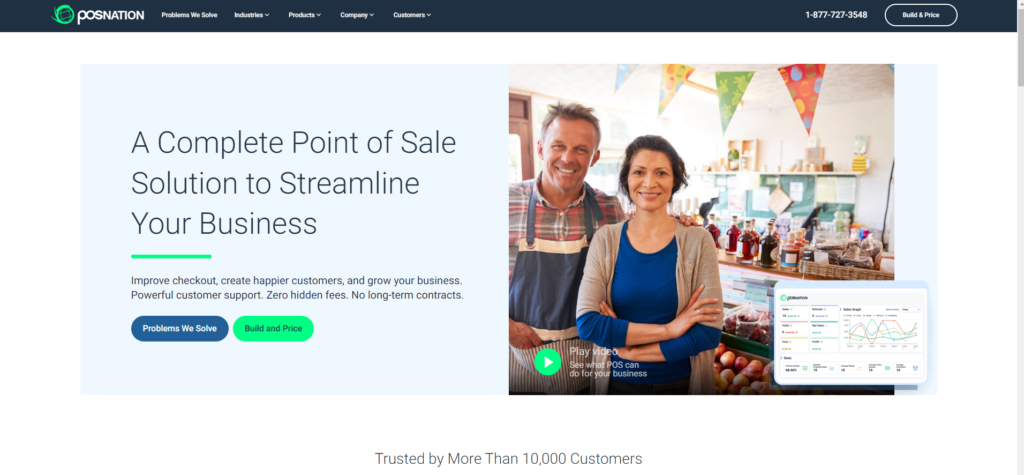This image is a screenshot of the POS Nation website. The logo, which resembles a green globe-like circular object, is prominently placed at the top. The website's header, styled in a dark blue color, contains several navigation tabs. Some of them, though slightly blurry, include "Company" and feature a contact phone number, 1-877-727-3548, displayed in the top right corner. To the right of the phone number is a potentially labeled button for "Build a Price."

The main body of the webpage has a staged photograph on the right side featuring a man and a woman. The woman stands with her arms crossed, and the man has his left arm around her shoulder. Both appear to be in a shop, possibly indicating their business. To the left of the image is compelling text that reads: "A complete point-of-sale solution to streamline your business. Improve checkout, create happier customers, and grow your business. Powerful customer support, zero hidden fees, and no long-term contracts."

Beneath this text are two action buttons—a blue one labeled "Problems We Solve" and a green one that says "Build and Price." At the bottom of the webpage, a testimonial states, "Trusted by more than 10,000 customers," reinforcing the credibility and trustworthiness of the service.